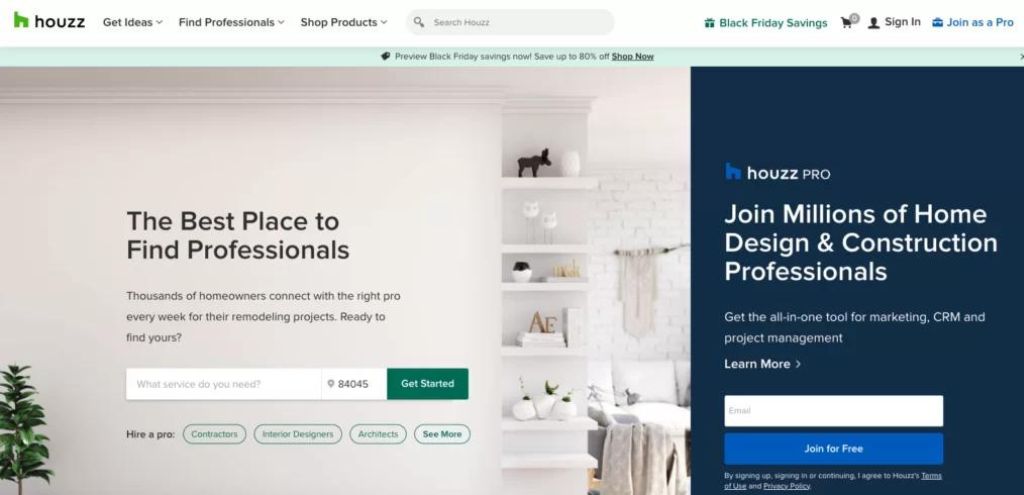The image showcases the Houzz website's header and a promotional section. The header features a green house icon resembling an "H" and "HOUZZ" written in black text. To the right, there are dropdown menus labeled "Get Ideas," "Find Professionals," and "Shop Products." A search bar, with a magnifying glass icon, is labeled “Search Houzz.” Further to the right, there are options for "Black Friday Savings," "Sign In," and "Join as a Pro." 

Below the header, the main section has a backdrop of a wall displaying overlaid text: "The Best Place to Find Professionals. Thousands of Homeowners Connect with the Right Pro Every Week for Their Remodeling Project. Ready to Find Yours?" Beneath this, there are input fields: one labeled "What Service Do You Need?" and another with a location pin showing "84045." A dark green "Get Started" button follows. The background includes shelves and a sofa, adding a homey touch to the scene.